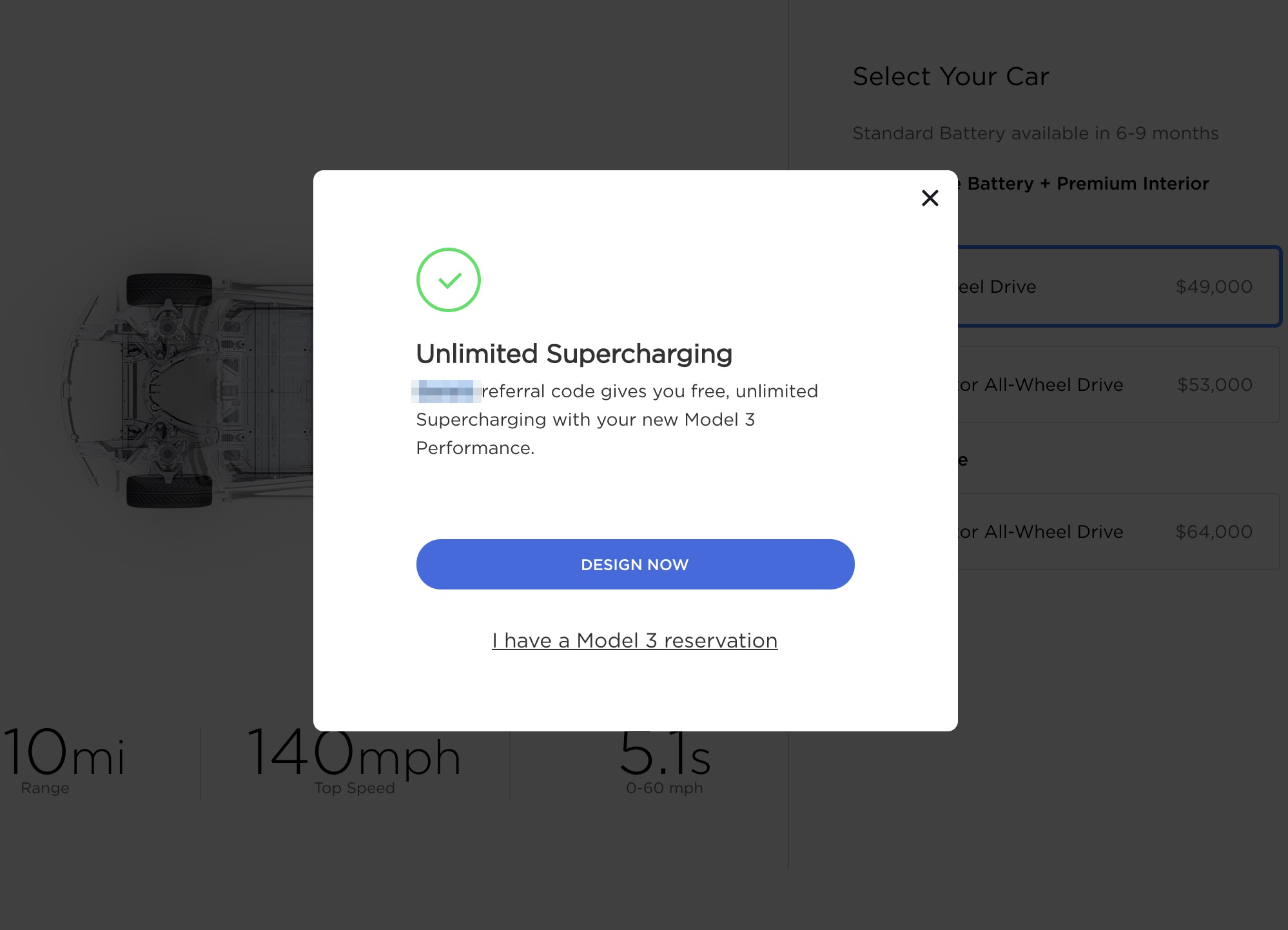Screenshot of a pop-up box related to Tesla supercharging. In the upper right corner of the box, there's a black "X" icon to close the pop-up. The middle portion features a green circle with a green checkmark inside it. Just below this, the text reads "Unlimited Supercharging" in prominent font. Beneath this, in black letters, it states "Blank refused to supercharge." The design includes a button below that, which says "Referral code gives you free unlimited supercharging with your new Model 3 Performance." At the very bottom of the pop-up, there is a statement saying "I have a Model 3 reservation." This pop-up appears in front of what looks like a Tesla page for owners, possibly part of the Tesla owner portal or a similar section on their website.